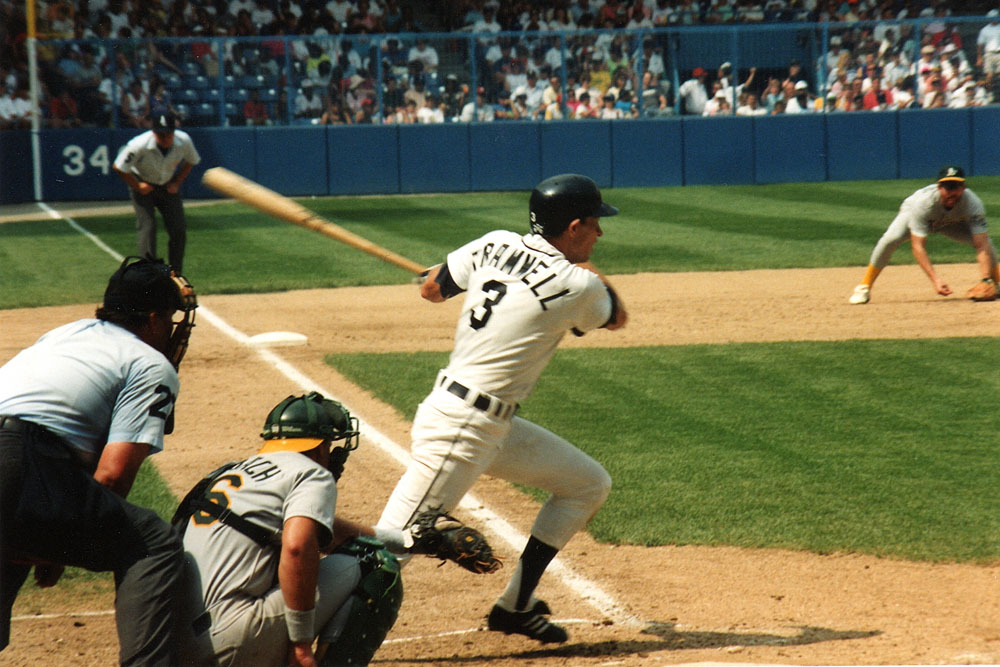This horizontally aligned, rectangular photograph captures an intense moment in a professional baseball game. In the heart of this outdoor scene, a player in a white uniform with the name "TRAMMEL" and the number three emblazoned on the back is on the verge of running after an impending hit. His front leg is pushed back diagonally while his back leg is bent, almost touching the ground. The tan bat pointed towards the top left corner signals his readiness to move. He dons a black hat, black belt, and black socks which complement his uniform's black lettering and trim.

To the right of him is another player in a gray and yellow uniform, leaning forward with legs broadly spread apart, seemingly poised for action. His hands are near the ground, emphasizing his alert stance. Further enhancing the scene is an umpire in the bottom left corner, garbed in a similar gray and yellow uniform with a green helmet, observing closely.

The background showcases a vibrant audience seated in sections divided by a long blue barrier. The crowd, dressed in hues of red, white, and various colors, spans the top portion of the image, adding energy to the setting. A white pole with an orange top and white bar is noticeable beside them, along with a chalk line and base cutting diagonally across the green grass and light brown dirt path of the field.

Foreground elements include a player squatting closely, in a light gray uniform with a green and yellow number six and a green arc labeled "CH" on the back, and another player donning a hat and white short-sleeve shirt, holding a mitt up by their face. The image captures the dynamic interplay of players and audience, transporting viewers into this high-energy baseball game.